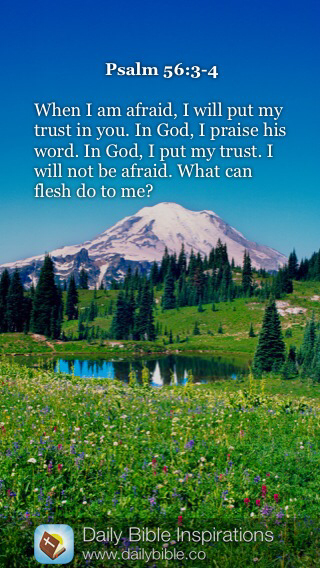The image is a collage with a graphic orientation, featuring a serene mountain landscape. The background is a vivid photograph of a snow-capped mountain under a clear blue sky, with a lush meadow full of wildflowers in various colors at its base. In the middle of the meadow, there's a tranquil mountain lake reflecting sporadic pine trees situated between the lake and the mountain.

At the top of the image, bold white text set against the blue sky reads, "Psalm 56: 3-4." Below this, in smaller white text, the scripture continues: "When I am afraid, I will put my trust in you. In God I praise his word. In God I put my trust. I will not be afraid. What can flesh do to me?"

At the very bottom of the image, overlaid on a slightly opaque black background, there is a logo of a Bible accompanied by text that says, "Daily Bible Inspirations" and the website "www.dailybible.co." The harmonious blend of nature and scripture creates an inspirational and calming visual.